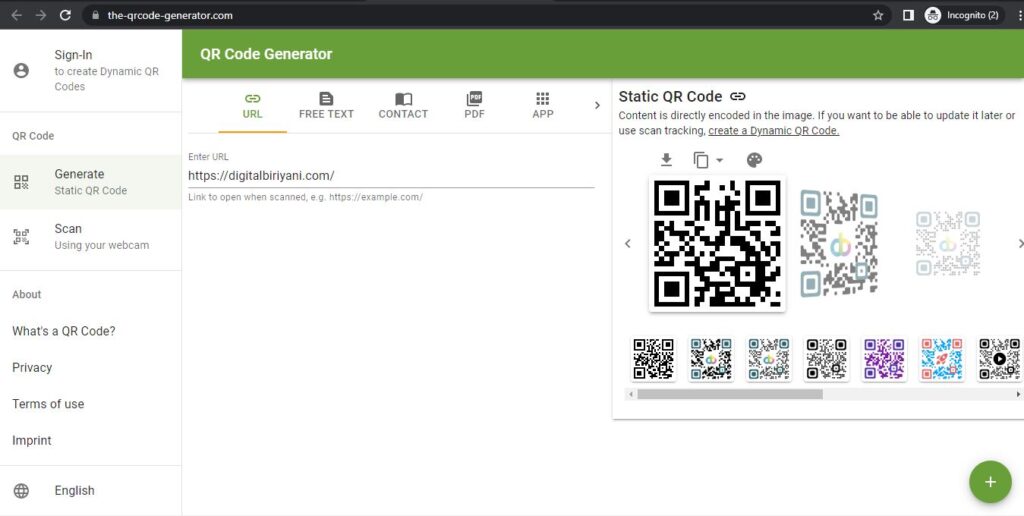Screenshot of a QR Code Generator Interface

The image is a detailed screenshot of a QR code generator webpage loaded in Google Chrome's incognito mode. The browser's address bar appears in black, distinguishing the private browsing session. The webpage interface prominently features a green header bar stretching across the top, emblazoned with the words "QR Code Generator" in white text. Directly beneath this header, in the page navigation area, the option "URL" is highlighted in yellow, signifying the currently active page for generating QR codes linked to URLs.

Below this navigation section, a succinct text box prompts users to "Enter the URL: https://digitalbriyani.com", highlighting the specific webpage intended for QR code generation. 

To the right, a sidebar menu provides additional functional options, including:
- Sign in
- Create a dynamic QR Code
- Static QR Code (selected option)
- Scan using your webcam
- And more options under headings like "What's a QR code?", "Privacy", "Terms of use", and a language selection feature set to English.

The central portion of the page elaborates on static QR codes, emphasizing that the content is directly encoded into the QR image and cannot be updated. Above this functional description, users can switch between generating QR codes for various data types, including free text, contacts, PDFs, and more through a dropdown menu.

Toward the lower part of the interface, numerous sample QR codes are displayed, illustrating different styles and formats. These sample codes are akin to the pixelated appearance of the iconic "missing number" graphic from Pokémon Red and Blue, providing a visual familiarity for visitors.

Additionally, the bottom right corner of the webpage features a prominent green circle with a plus sign, likely representing a quick-access button for generating new QR codes. This comprehensive interface affirms the versatility and functionality of the QR code generator tool.